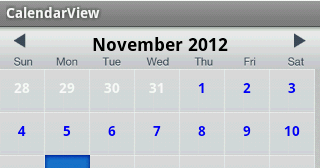This is a detailed screenshot of a calendar application displaying the month of November 2012. At the very top, a dark gray bar spans the image, and in white font, it reads "calendar view." The calendar itself is a light gray, providing a subtle contrast against the black font indicating "November, 2012." Flanking this text are arrow symbols, allowing for navigation between different months.

The calendar grid is labeled with the days of the week: Sunday, Monday, Tuesday, Wednesday, Thursday, Friday, and Saturday. The preceding days from October—28th, 29th, 30th, and 31st—are shown in white font under Sunday, Monday, Tuesday, and Wednesday, indicating they are part of the previous month.

November starts on a Thursday, marked with the 1st in blue font, as are all the subsequent dates of the month displayed. Progressing in sequence, the calendar shows Thursday, the 1st, Friday, the 2nd, Saturday, the 3rd, followed by the week starting with Sunday, the 4th, and ending with Saturday, the 10th. The detailed view of the calendar stops at this point, providing a snapshot of the early part of November 2012.